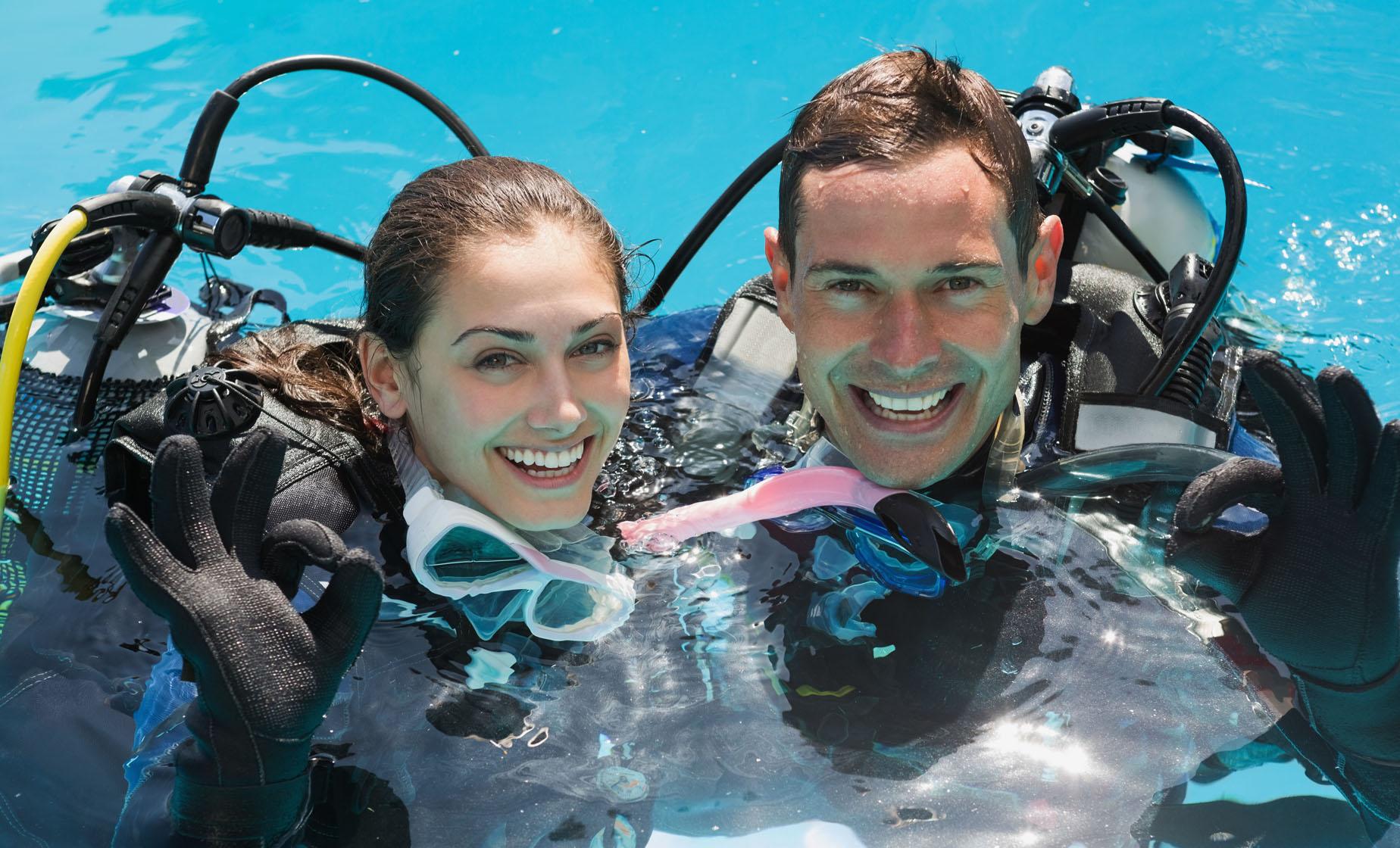A vibrant photo captures a young man and woman, probably in their 20s, posing happily in crystal blue water with the sun reflecting off the surface, giving it a bright, almost white appearance. Both are in black scuba diving gear, with tanks on their backs and tubes hanging out. Their hair is dry, suggesting they are about to dive rather than having just emerged. On the left stands the woman, her dark hair pulled back into a sleek ponytail, revealing her smiling face with goggles around her neck. She has a black glove on and holds up her right hand in an "OK" sign. On the right is the man, with short dark hair, a high forehead, and a wide smile, mirroring the woman's pose by holding up his left hand in an "OK" sign, also wearing black gloves. Both divers are enthusiastically looking straight at the camera, capturing a moment of excitement and readiness. Notable details include one of the woman's tanks having a yellow hose, while all of the man's hoses are black. The scene is devoid of any underwater life, focusing entirely on the joyful expressions and camaraderie of the two divers.